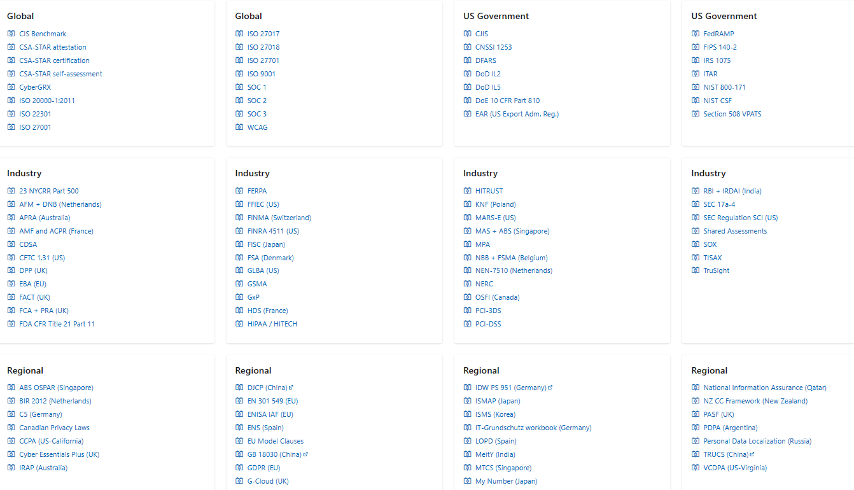The image is a screenshot featuring diverse categorization of various names. These names are organized into distinct columns and rows. The top row includes labels such as "Global" and "U.S. Government," repeated twice. The second row is exclusively labeled "Industry," repeated four times across its columns. The final row is labeled "Regional" across all columns. Within these categories, some of the entries appear as acronyms or codes. For example, in the second row of the last column, the acronym "SOX" is visible, and in the first row of the third column, the acronym "CIS" appears.